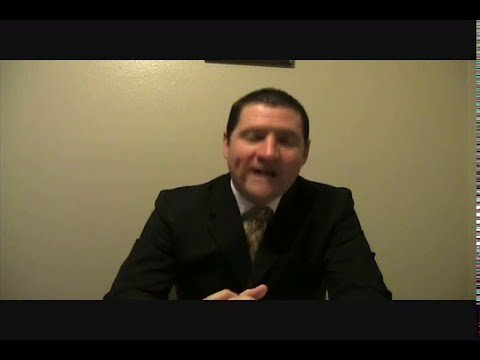The image depicts a gentleman speaking, likely captured during an online interview or video call, suggested by the framing that resembles a screenshot. The man is seated at a dark table, centrally positioned in the image. He has very short, dark hair cropped close to his scalp and above his ears, and he appears to have a light or possibly Hispanic skin tone. His eyes are closed mid-speech, emphasizing a moment in motion, with his mouth open and hands visible in front of him. His face is round and full with a broad, straight nose and a notable dimple in his right cheek (left from the viewer's perspective). He is dressed in a black suit with a white shirt and a tie of tan mixed with greenish-brown hues. The background is plain, featuring an off-white or cream wall with a slight light source over his right shoulder. The image's overall dark tone may affect the color accuracy. Additionally, the frame includes thin black stripes at the top and bottom, bordered by thicker, lighter black strips.